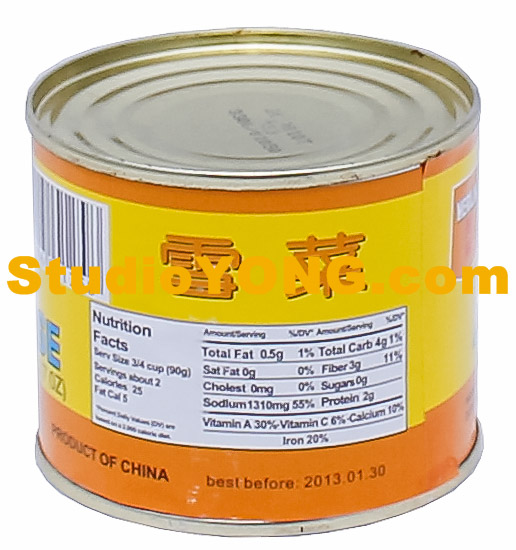This color photograph displays an up-close view of a small, silver metal can with an orange and yellow label, bordered by a clean white frame. The label features a prominent orange border at the top and a wider orange border at the bottom. The central section of the label is yellow with Chinese characters written in orange, and the right side exhibits a barcode. Overlaid in yellow text is the URL "studioyong.com," positioned across the label area, blending into the yellow background. The nutritional facts are detailed in a white rectangle with black text, listing serving size as three-fourths cup (90 grams), totaling approximately two servings per container, with 25 calories and 5 from fat. At the bottom of the label, in bold black letters, it states "Product of China," followed by "Best Before 2013.01.30" in lighter black print.